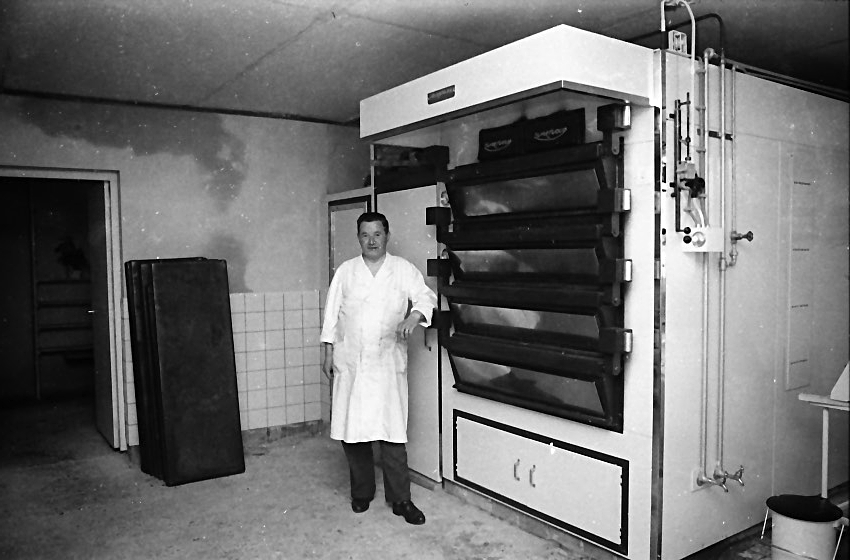The black-and-white vintage photograph captures a man in his mid-thirties with short black hair, wearing a long white coat, dark pants, and black shoes. He stands slightly to the right of the center of the image, leaning with his left elbow on a large, white metal baker’s oven that dominates the background. The imposing oven, towering approximately 12 feet tall, features four black glass doors lined at the bottom and is accompanied by an exhaust apparatus protruding from its top. The oven side shows an intricate network of pipes, electrical conduits, and valves, suggesting its industrial nature. To the side of the oven, there is a bucket and further plumbing fixtures. The room has a stark, utilitarian appearance with tiled lower walls and a plain concrete floor, reflecting the era's functional design. The left side of the image reveals an open doorway leading into an unseen space, with the overall ambiance giving a glimpse into a bygone era of industrial labor.